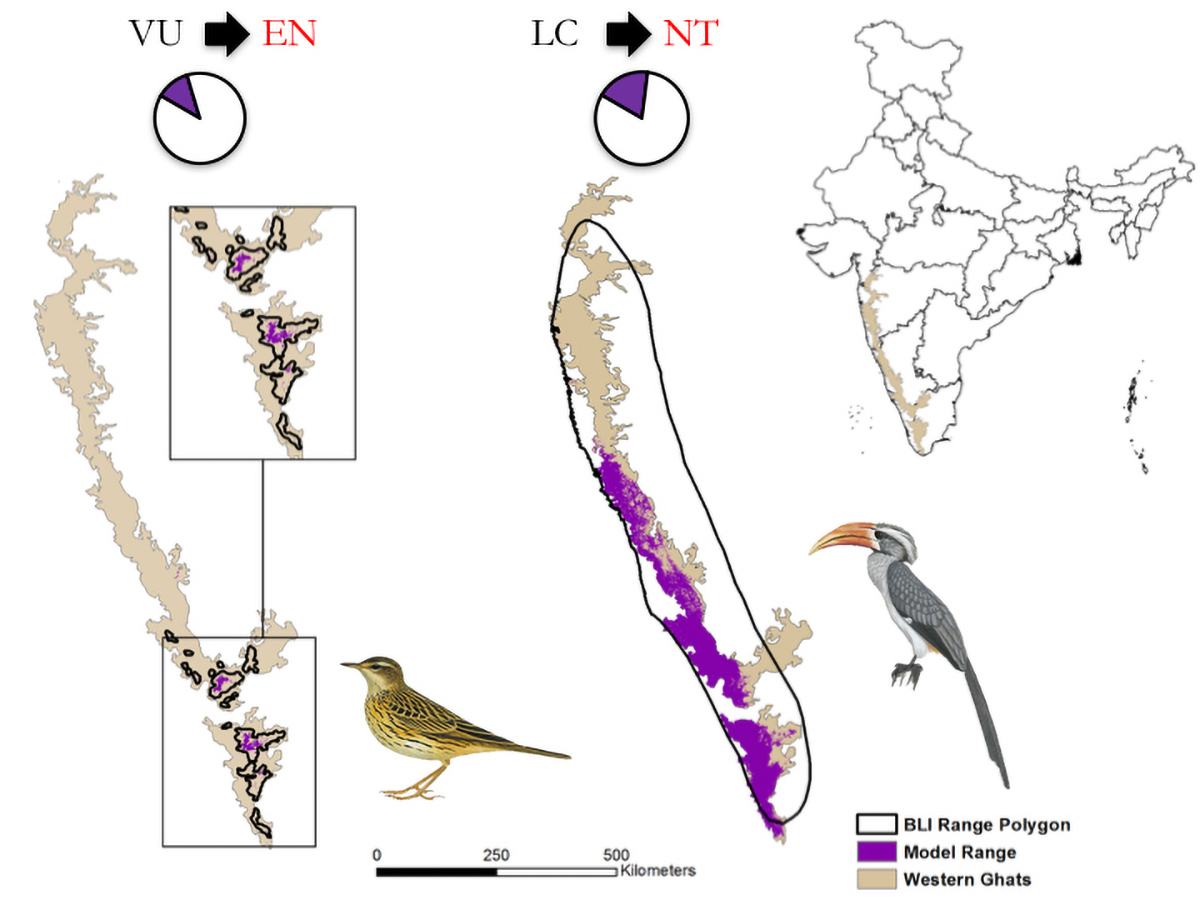The image is a detailed visualization of a threat assessment map for two bird species, overlaid on a world terrain map to illustrate their ranges. The central aspect features a yellow and black bird and a gray and white bird with an orange beak. The map highlights the areas these birds inhabit, using white to represent BLI range polygons, purple to indicate model ranges, and beige for the Western Ghats landmass.

In the bottom right section, there is a detailed legend: "BLI range polygon" in white, "model range" with a purple box beside it, and "Western Ghats" indicated by a tan square. Additionally, a country on this map is encircled and shows parts shaded in purple, denoting specific regions, while another country includes two inset squares showing zoomed areas marked with black circles and purple shading.

The left side of the image contains the map corresponding to the yellow and black bird, featuring a pie chart with about one-eighth in purple and the rest in white, labeled with "VU" leading to an arrow pointing to "EN". Below the chart, the map highlights a small portion in purple indicating where this bird lives or migrates. 

Similarly, on the right side, a gray and white bird with an orange beak is shown alongside a larger map and a corresponding pie chart that reveals a larger purple section, labeled "LC" with an arrow pointing to "NT". Both pie charts offer a visual percentage assessment of the bird's threat levels.

Additionally, the map includes a key indicating distances of 0, 250, and 500 kilometers per inch. Each section of the map is meticulously labeled, providing a comprehensive overview of the birds' habitats and the respective threat assessments.